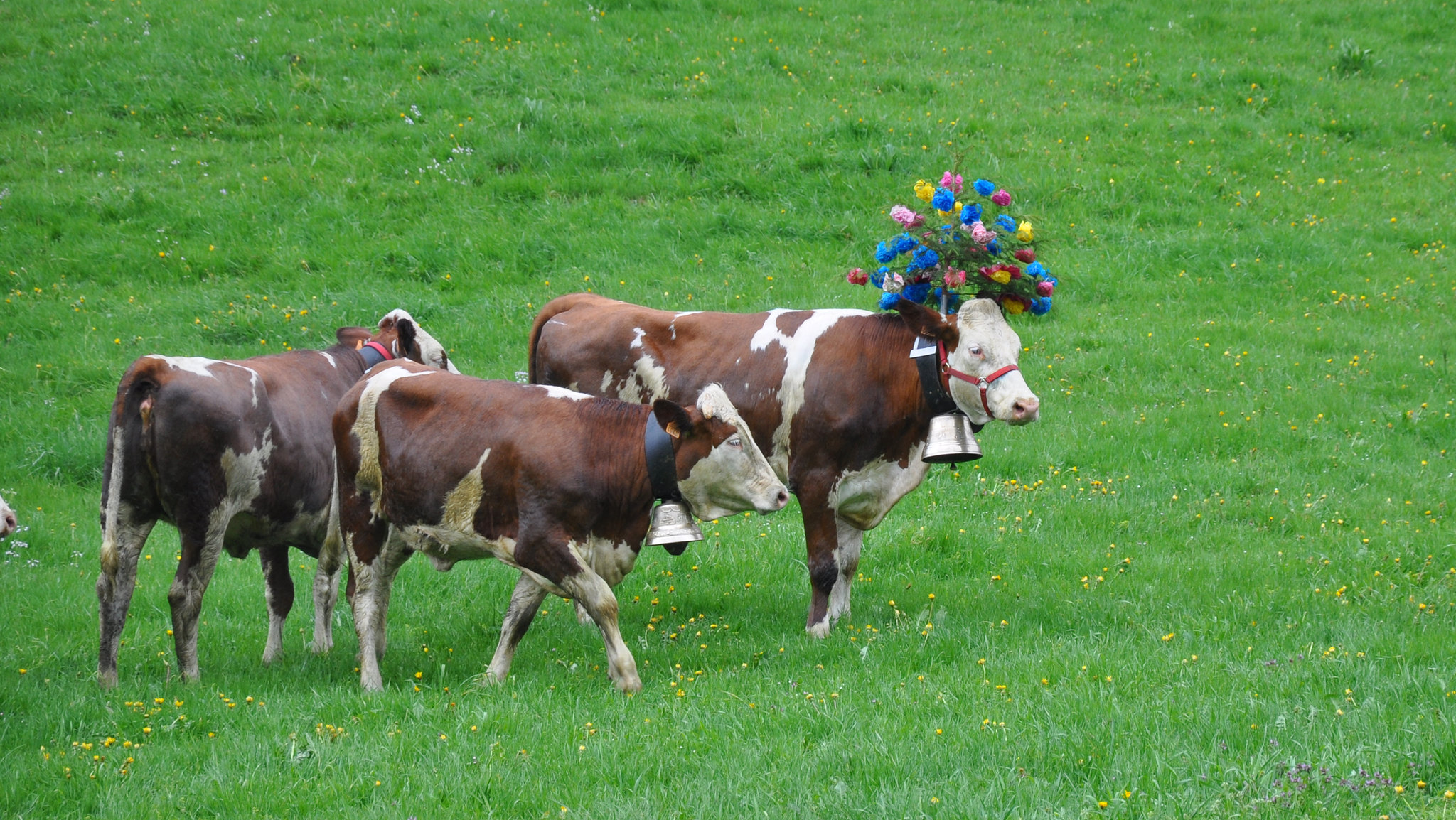In this vivid outdoor photograph, three spotted cows stand together in a lush, vibrant green pasture dotted with small yellow flowers. The cows, primarily brown with contrasting whitish faces, legs, and tails, all have silver bells hanging around their necks. Two cows face to the right, with one positioned centrally and the other beside it, while the third cow looks away from the camera. The cow in the middle stands out with a bright, colorful bouquet of blue, pink, yellow, and red flowers attached to a red halter on its head, adding a decorative touch to the serene pastoral scene.